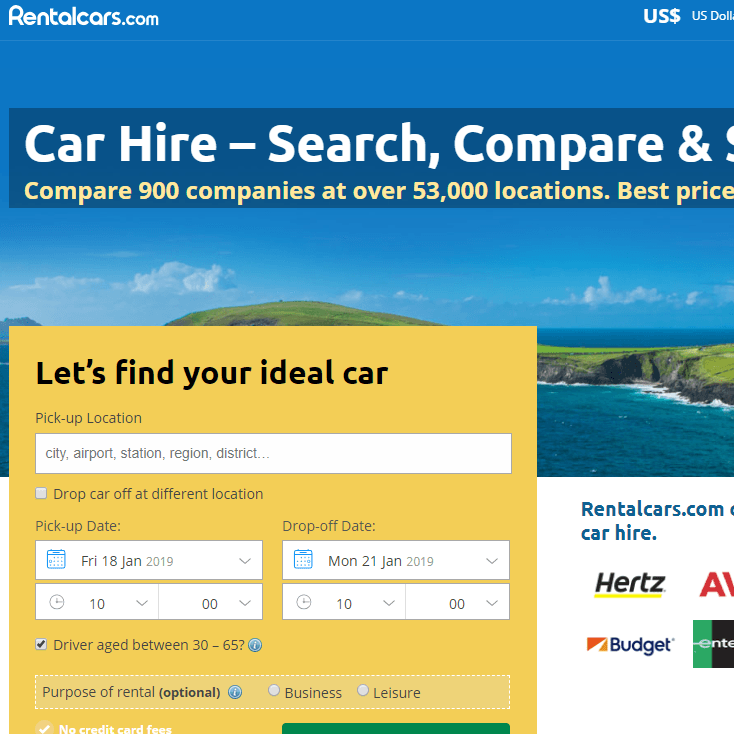The webpage for rentalcars.com features a serene, bucolic image as its backdrop, depicting a peninsula covered in green foliage and rocky terrain, flanked by tranquil waters on both sides under a partly cloudy sky. Superimposed on this idyllic scene is a rectangular overlay containing various informational elements. 

At the top of the overlay, "Rentalcars.com" is prominently displayed with a capital 'R.' Adjacent to it, the currency is indicated as "US dollars (USD)," though 'dollars' is partially obscured, showing only "D-O-L-L." Below this, a navy blue rectangle with bold white text declares, "Car Hire - Search, Compare &," though the subsequent text is cut off.

In smaller, yellow text just beneath, the offer to "Compare 900 companies at over 53,000 locations. Best price." encourages users to explore competitive rates. Another gold-colored box further invites interaction with the prompt, "Let's find your ideal car," inscribed in black font.

Interactive input fields allow users to enter details such as the pickup location, pickup date, drop-off date, and whether to drop the car off at a different location. Options for the driver's age range (30 to 65) and the purpose of the rental (business or leisure) are provided through checkboxes and clickable circles, respectively, ensuring a customizable search experience.